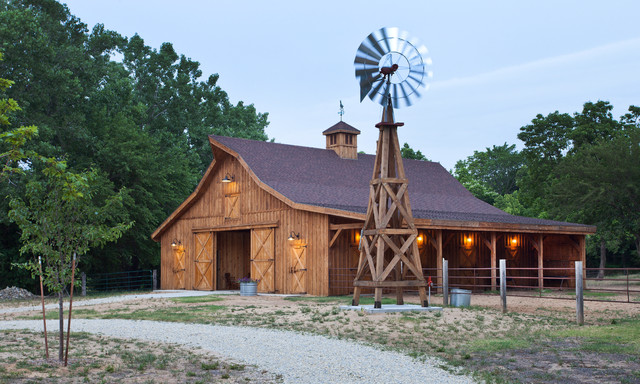The photograph captures a large, two-story wooden barn situated on a plot of land with sparse, dead grass interspersed with dirt. The barn, comprising vertical wooden panels and a shingled roof, features open large wooden doors that provide a glimpse inside, though no distinct interior details are visible. A gravel path leads straight to the entrance and then curves off in one direction in front of the barn. Surrounding the barn is a wooden fence, possibly intended for horses, and the area is encircled by numerous trees. 

In the foreground stands a freshly planted baby tree, supported by a couple of poles to help it grow upright. Adjacent to the barn, a tall, T-shaped wooden structure supports a large, silver windmill, spinning and seeming almost as tall as the barn itself. This windmill is mounted on a concrete slab and includes a water spigot with a red handle nearby. Additionally, a corral with what might be horse stalls extends behind the barn. On the roof of the barn, there is a small chimney-like protrusion that features windows and is topped with a weather vane, completing the pastoral scene under a clear blue sky.